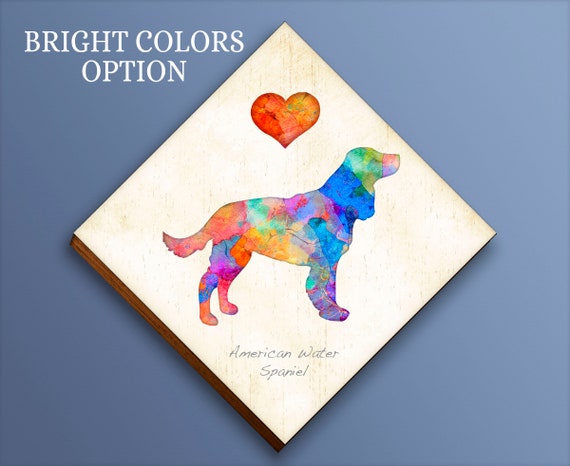The image depicts a wooden picture board, intricately designed in a square shape but oriented as a diamond. The background is a serene bluish-gray hue, providing a calm backdrop for the vibrant artwork featured on the board. At the top, bold text reads "Bright Colors Options," hinting at the vivid palette used in the image. The focal point of the board is a colorful dog, specifically labeled as an "American Water Spaniel" below the image. The dog is rendered in an array of bright colors, including orange, blue, green, red, and purple, giving it a lively and dynamic appearance. Above the dog, a multi-colored heart, predominantly in shades of orange with specks of green, adds an extra touch of warmth and affection to the composition.